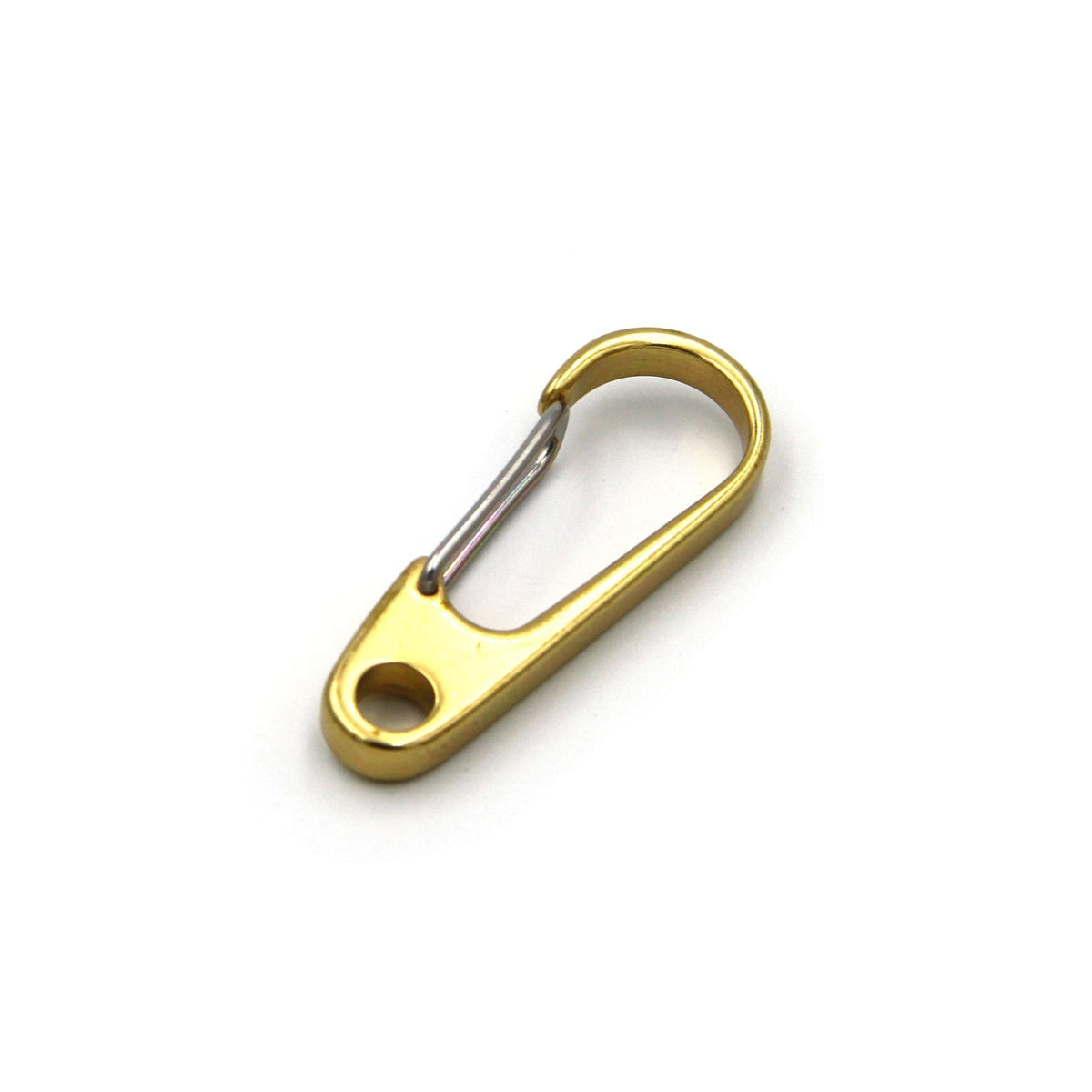The image displays a small, decorative carabiner set against a pure white background with a subtle light gray drop shadow. The carabiner, made of a golden or brass-colored metal, has a thin, tapered frame with a rounded bottom that extends upward and curves into an upside-down U or C shape. The main body features a large hole at the base, likely for attachment purposes, and the left side incorporates a stainless steel spring mechanism, enabling the clasp to open and close securely. Positioned at a diagonal angle from the bottom left to the top right, this carabiner's ornamental design and delicate build suggest it is not intended for heavy-duty use or extreme sports.